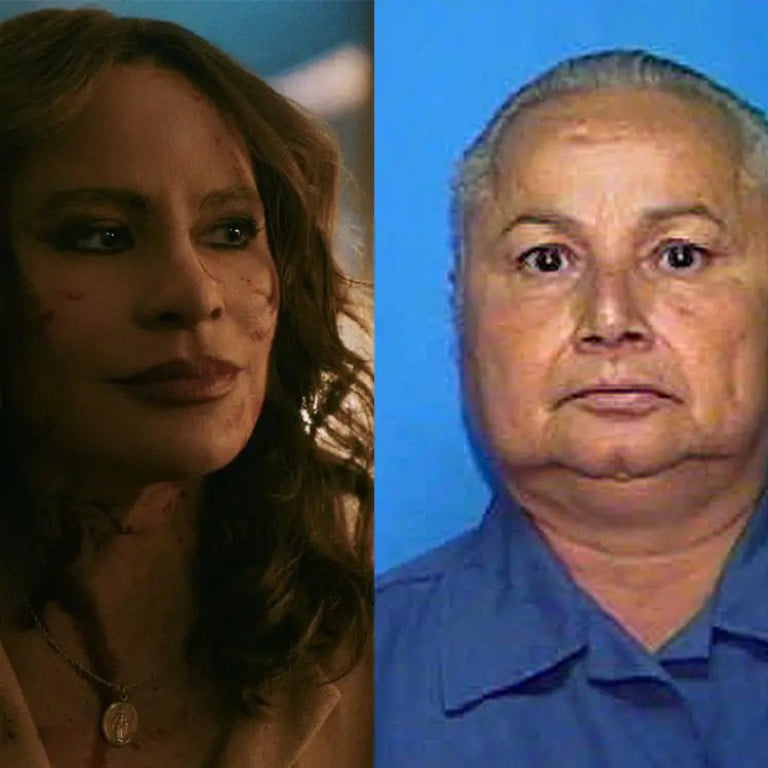The image depicts two people against a bright turquoise background. On the left, there is a woman with brown hair and striking red lipstick, accessorized with a gold necklace. Her face appears to have bloody red markings, and she is gazing slightly to the right. On the right is a man with brown eyes, wearing a blue collared shirt. He looks directly at the viewer with wide, somewhat fearful eyes. His image appears blurrier compared to the woman's, giving it a less focused appearance. The scene evokes an intense and unsettling atmosphere, reminiscent of a mug shot.